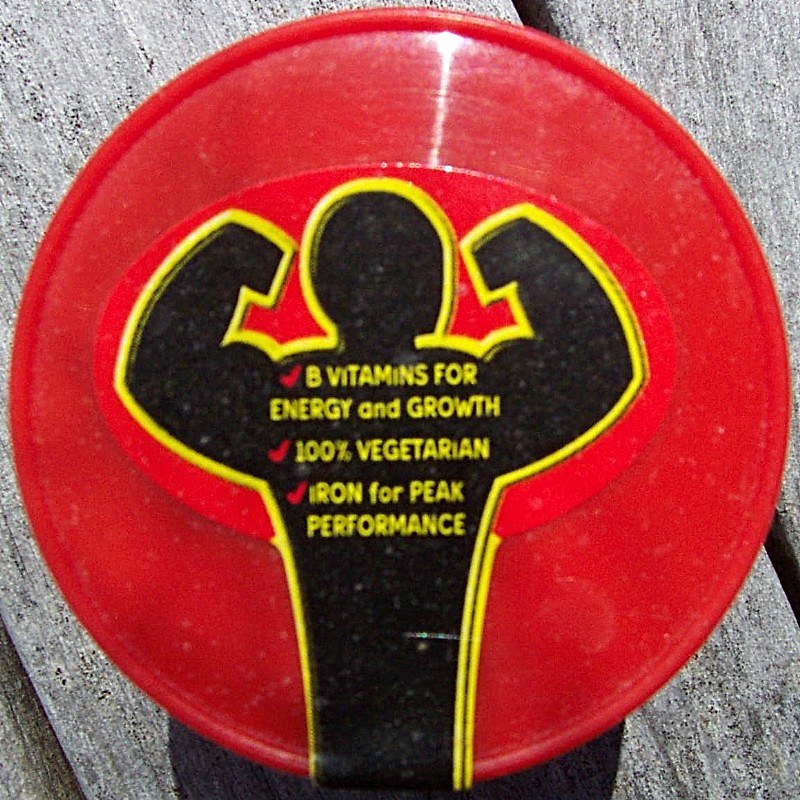The image features a red frisbee viewed from above, resting on a grayish wooden table with visible slats. At the center of the frisbee is an oval sticker. The sticker depicts a muscular man in black, outlined in yellow, flexing his arms. Below the figure, the sticker includes three red check marks with the following text: "B vitamins for energy and growth," "100% vegetarian," and "Ironed for peak performance."